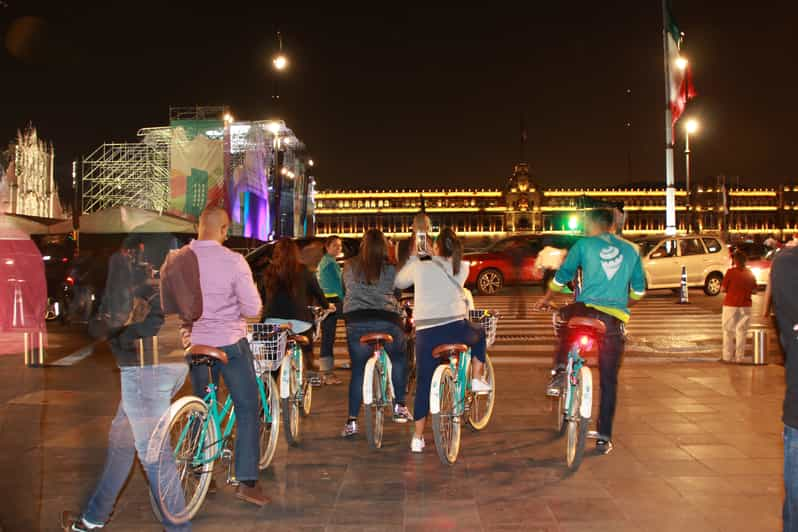This nighttime photograph captures a busy urban scene with a group of around 5 to 6 cyclists gathered on a brown-tiled walkway, waiting at a large crosswalk. The cyclists, who appear to be tourists, are riding matching green bicycles with brown leather seats and white fenders, suggesting they are rentals. The scene is illuminated by streetlights, and the dark black sky above enhances the vividness of the lights. In front of the cyclists, various cars pass by on an asphalt road. The background features a long, wide building, strikingly outlined with yellow lights on its three levels, creating a rectangular shape with a prominent tower-like entrance. To the left, another building with banners and additional lights adds to the vibrant, bustling atmosphere of the cityscape. A person walking past appears ghostly and transparent due to the photograph's exposure.